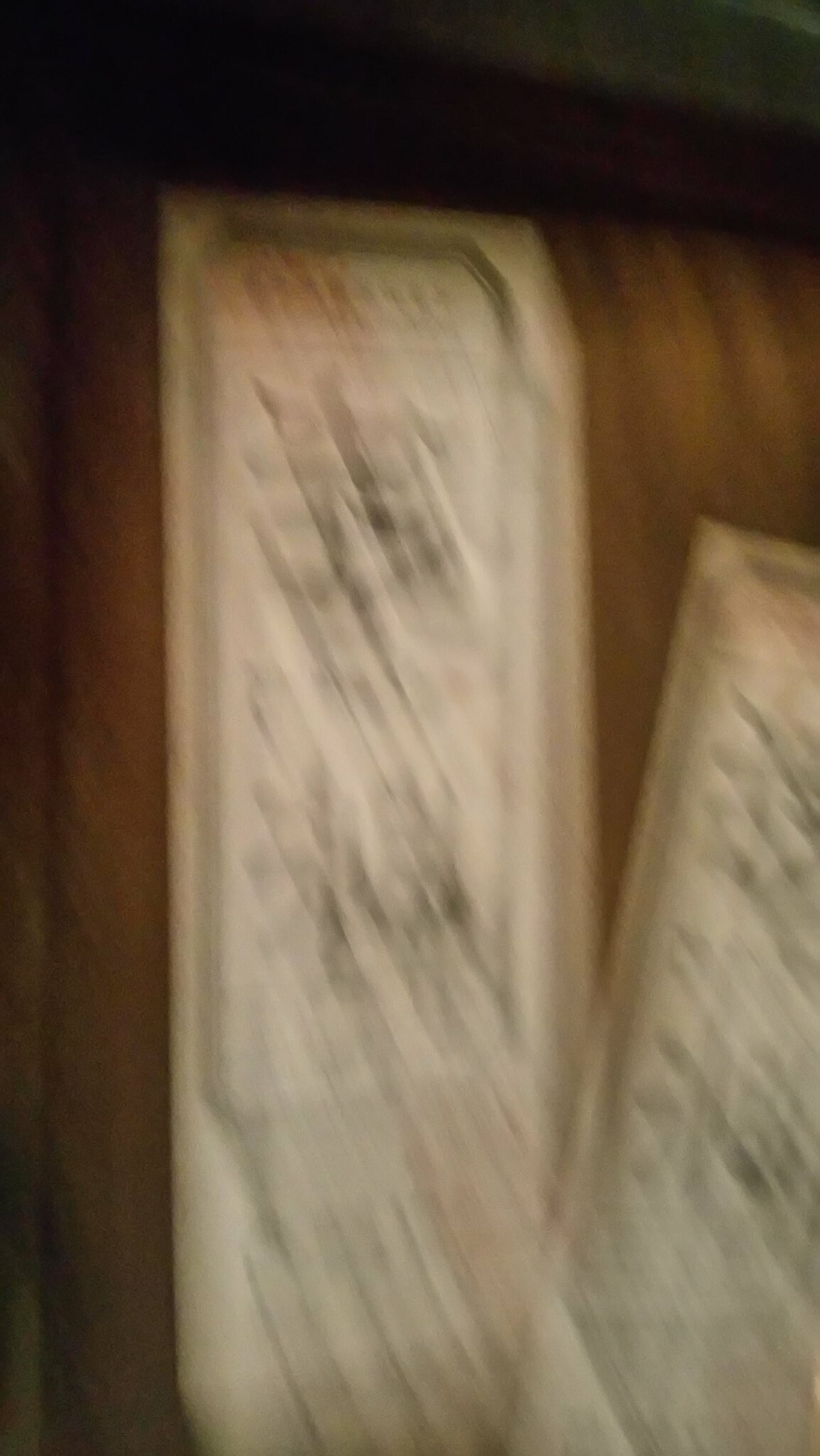In this very blurry photograph, we see two narrow, rectangular white slips of paper, each with black writing on them. These slips resemble tickets or receipts and feature a silver rim around their edges. The writing on the tickets appears to be Asian characters, most likely Chinese, and covers about three-quarters of the space within the long rectangular border on each slip. Despite the blur, it is discernible that the text was probably painted on with a brush. One of the tickets shows almost fully, while the other is slightly folded at the bottom and partially obscured. Both tickets seem to have some kind of ribbon hanging off one edge. They appear to be lying on a wooden table, with the background fading from black at the top to a medium brown towards the bottom. The blurriness of the image suggests it might have been taken in motion or due to a dropped phone, adding a dynamic, almost shadowy quality to the dark black writing against the white slips.